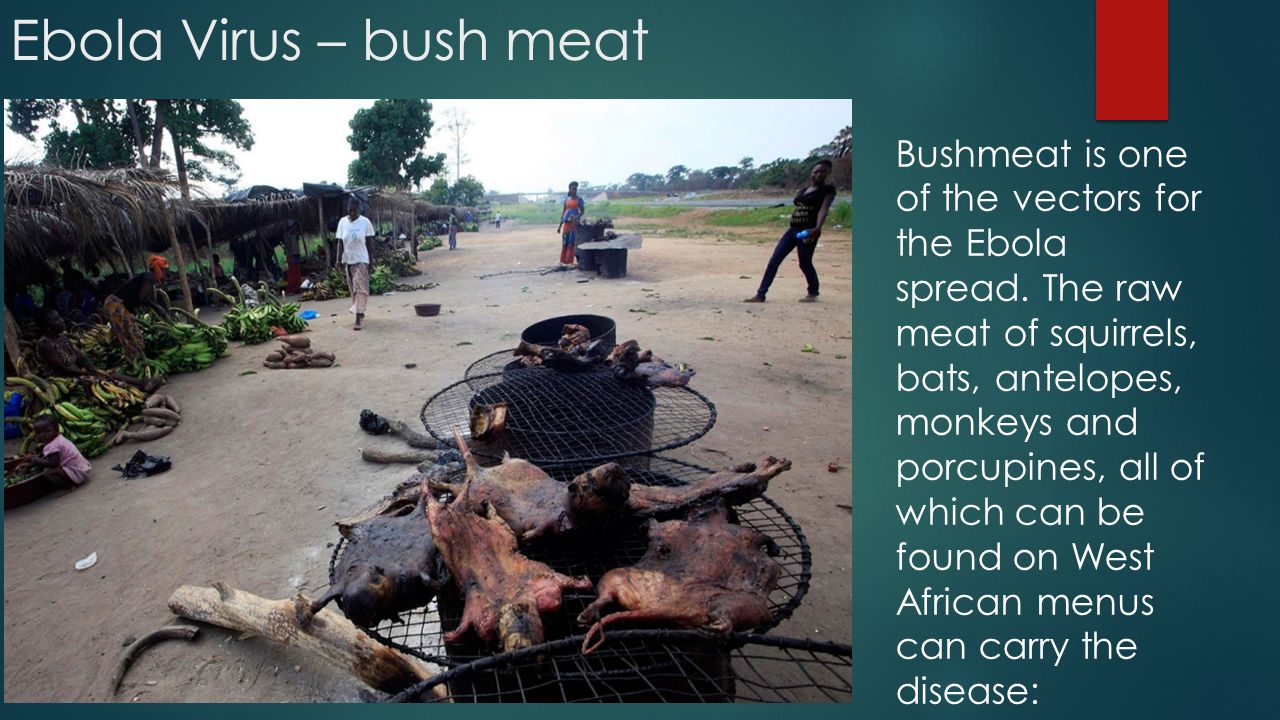The image prominently features a blue background with white text at the top stating "Ebola Virus = Bushmeat." On the right side, it further explains that "bushmeat is one of the vectors for the Ebola spread," highlighting that the raw meat of squirrels, bats, antelopes, monkeys, and porcupines—all common in West African cuisine—can carry the disease. The main visual component of the image shows a busy outdoor market scene. Several grills, fashioned from round wire racks placed on barrels, are cooking various animal carcasses on a dirt ground. People are seen walking around the market, where there are also piles of green bananas and possibly potatoes. In the background, there are multiple huts with brown, leafy tops amidst green bushes, plants, and trees. The sky appears white, and the overall scene captures a typical bustling West African market environment.